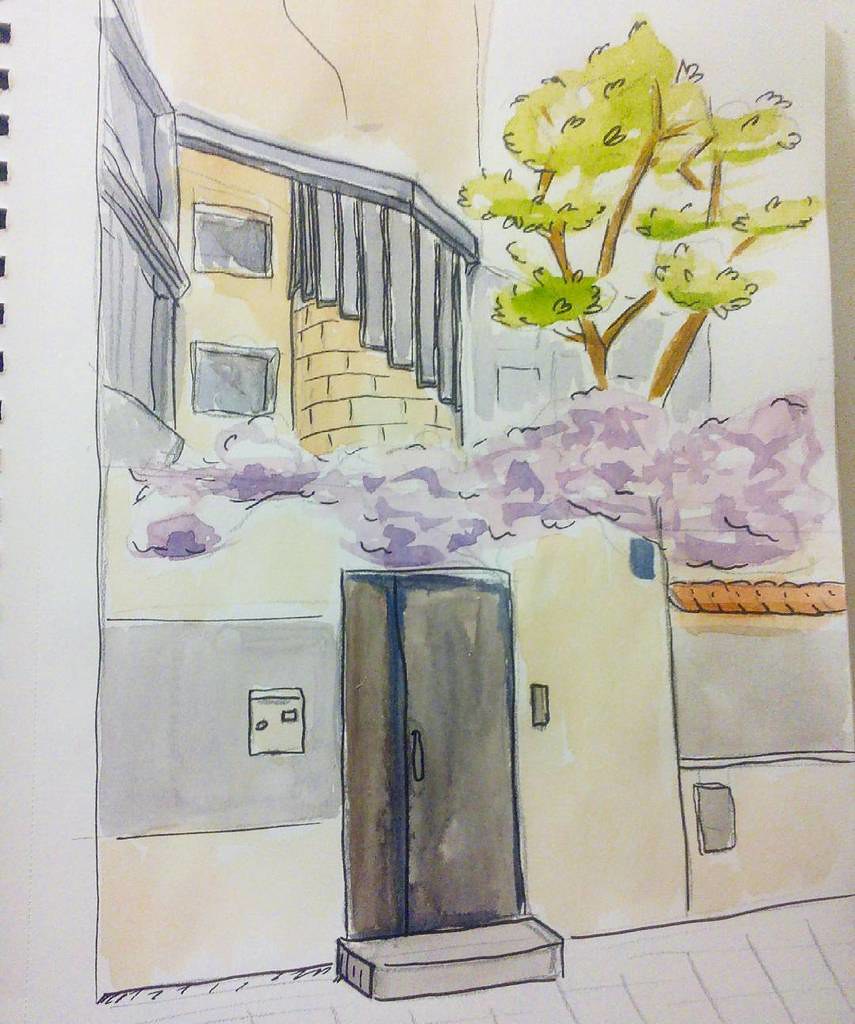This image is a photograph or possibly a scan of a delicate watercolor painting, rendered with bright yet gentle pastel colors. The central focus is a building featuring a dark gray door with a small matching step leading up to it. Just to the left of the door, a box—presumably a mailbox—is depicted. Above the door and its immediate surroundings, a soft gradient of light violet or purple shading adds a unique ambiance to the scene. The painting's hand-drawn characteristics are evident, especially along the edges, which appear to be part of an artist's notebook, dispelling any notion of it being AI-generated. Above the violet shading, a series of spiraling stairs ascend to an upper area, suggesting the presence of a balcony or another section of the tan-colored building. In the upper right-hand corner, a small tree emerges behind and possibly above the structure, adding a touch of nature to this quaint, charming setting.